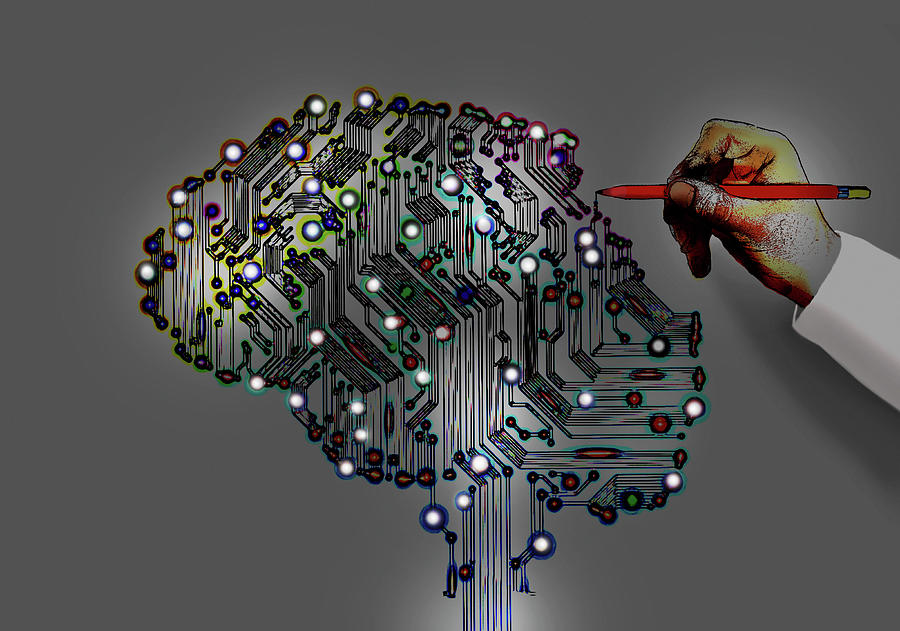In the center of the image, there is a detailed, digital-looking brain illustration, reminiscent of a circuit board with a complex network of black lines and white dots that give it a high-tech appearance. The brain is oval-shaped, with intricate circuitry patterns filled with various colors including light blue, green, yellow, red, and orange. This circuit-like brain design, imbued with a sense of electronic intricacy, stands out against a gradient background that transitions from dark gray to light gray.

Extending into the image from the right side is an illustration of a hand that appears to be holding a red pencil, poised to draw or interact with the digital brain. The hand, displaying a mix of colors—light yellow, white, orange, and sprinkled with purple dots—suggests a sense of shadow and depth. The fingers are gripping the pencil firmly, with a white sleeve visible over the wrist.

Overall, the detailed illustration seamlessly combines elements of human creativity and digital technology, with the hand and pencil artistically contributing to the structure of the brain, portraying a compelling synthesis of analog and digital realms.